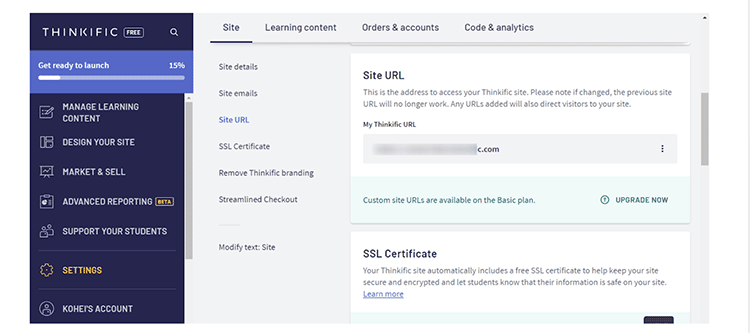Screenshot of a Thinkific Website Navigation Panel

This screenshot captures a section of a Thinkific website's admin interface, prominently displaying various navigational options for site management. The left-hand panel lists a series of configurable items including Site Details, Site Emails, Site URL, SSL Certificate, Remove Branding, Streamline Checkout, and Modify Text. The current selection is set to "Site URL", which is highlighted. On the right side of the window, detailed information about the Site URL is shown. It provides the current web address used to access the site and includes a cautionary note stating: "Please note if changed, the previous site will no longer work." This message emphasizes the importance of the URL configuration and its impact on site accessibility. The interface is clean and user-friendly, designed to provide administrators with easy control over critical aspects of their Thinkific websites.